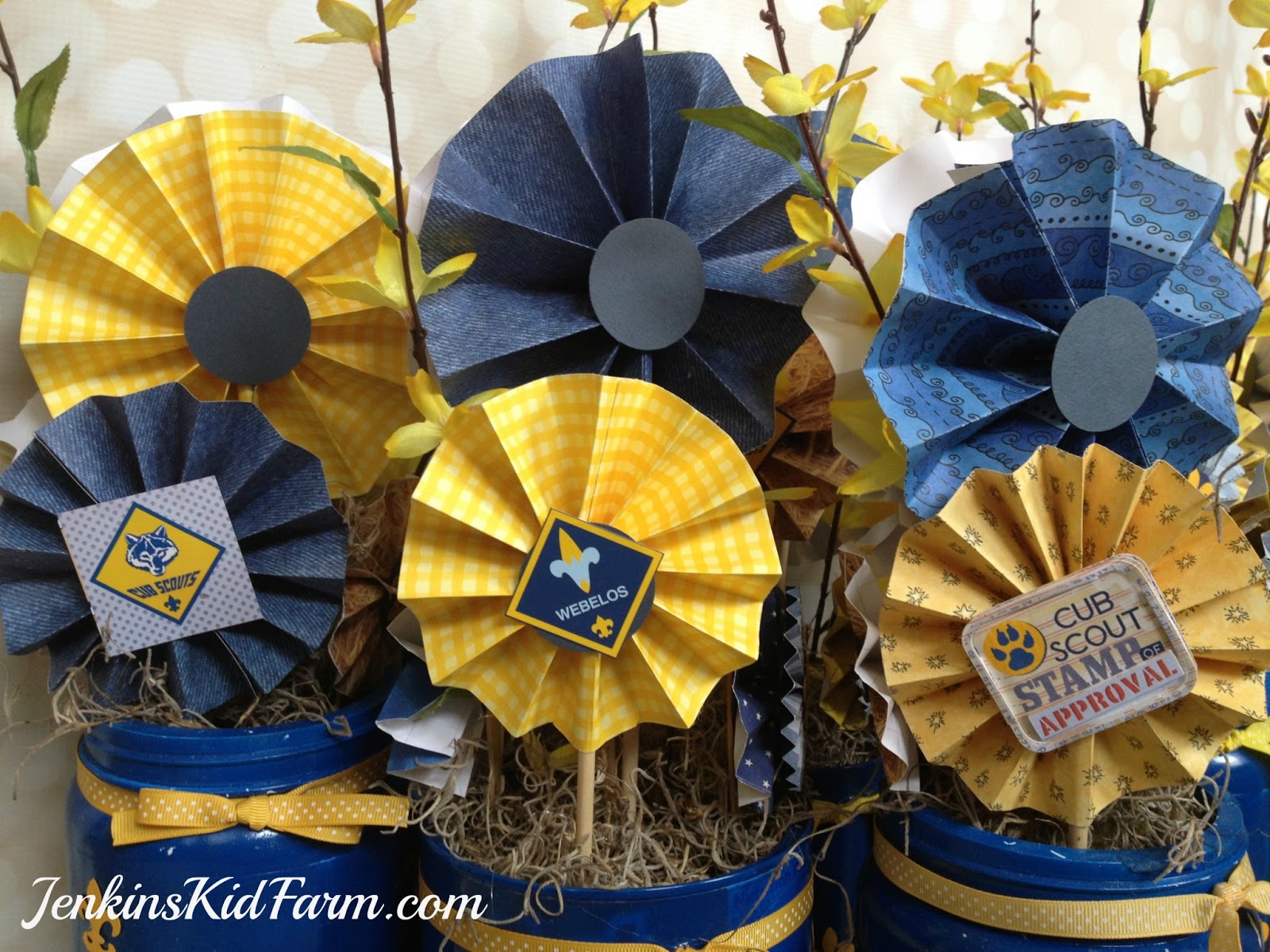This color photograph captures several bright blue flower pots adorned with yellow bows tied around the top rims. Each pot is filled with decorative elements and plant life, with the interiors stuffed with straw. Sticks placed inside the pots hold paper flower-shaped fans or pinwheels; there are six in total, evenly split between blue and yellow colors. The arrangement of these pinwheels features three at the back (yellow, blue, blue) and three at the front (blue, yellow, yellow), each of varying heights to ensure visibility. Notably, some of the pinwheels have stickers—specifically, one on the bottom left says "Cub Scouts," the front middle says "W-E-B-E-L-O-S," and the bottom right pinwheel bears the "Cub Scout Stamp of Approval." In the lower left corner of the photo, “JenkinsKidFarm.com” is visible in white text. There are no people present in the image, focusing the viewer's attention entirely on the vibrant, detailed art project.